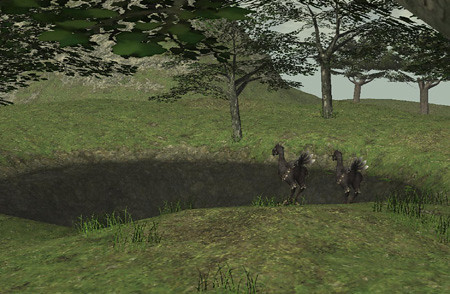The image appears to be a screenshot from a video game, likely the MMORPG Final Fantasy XI. The scene features a green area with polygonal trees that have a somewhat outdated design, indicative of older game graphics. In the middle of this green expanse, there's a small pond, with a mountain visible in the background to the left. The sky above has an unnaturally gray hue, further emphasizing the digital nature of the scenery.

Prominently in the foreground are two black or gray chocobos—bird-like creatures known from the Final Fantasy series, typically yellow but here shown with white-tipped tail feathers. These chocobos are gazing into the distance across the pond. The overall look of the image, including the stretched and unnaturally textured trees, suggests it may not be from a high-end game but rather an older title or one with lower graphical fidelity, reinforcing the likelihood of it being Final Fantasy XI.